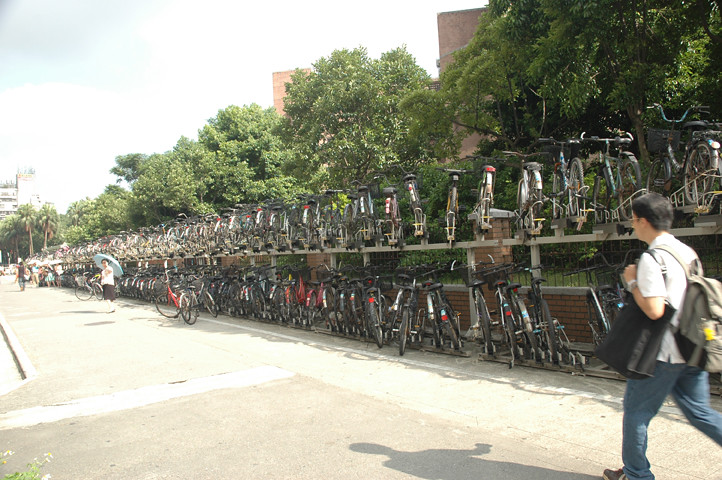The image captures an extensive bicycle parking area lined along a red brick wall. The parking setup features two levels of bikes, with some parked on ground level and others elevated about a foot above. This forms a continuous, almost endless line of bicycles stretching far into the distance from the right side towards the middle left of the photo. A young man in a white t-shirt, blue jeans, and carrying a green or gray backpack with a yellow detail is walking on the right side, holding a black rectangular object under his left arm. Further into the distance is a person with a blue umbrella, wearing a white t-shirt and black shorts, though they are slightly overexposed. The scene is framed by a row of broadleaf trees behind the brick wall and a wrought iron fence interspersed between the bricks. Some red brick buildings are faintly visible behind the trees. The bright sky overhead fades to white, while the overall scene creates a bustling yet orderly atmosphere.